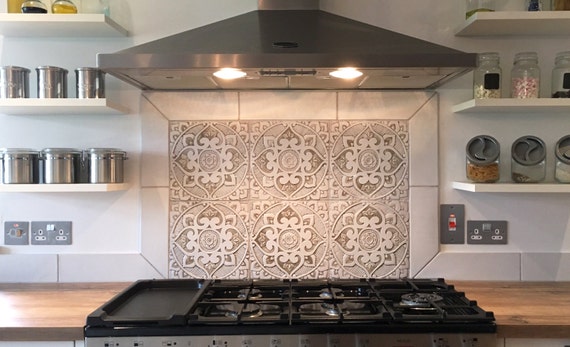This color photograph captures a detailed close-up of a kitchen stovetop range set into a large butcher block countertop. The stovetop is black with four silver gas burners, accompanied by an additional griddle on the left end. Above, a sleek range hood with a black top and silver bottom features two white lights illuminating the area below. Flanking this scene are symmetrical arrangements of white shelves on either side. The left set of shelves holds three rows of silver containers and small rounded glass bowls resembling candles at the top. On the right, the shelves display clear glass containers sealed with gray covers, and additional jars of unknown contents. The backdrop features an intricate mosaic of tan and cream tiles, with central circle designs akin to a four-petaled flower in dark gray or black tones, emphasizing a stylish and sophisticated ambiance in the kitchen.